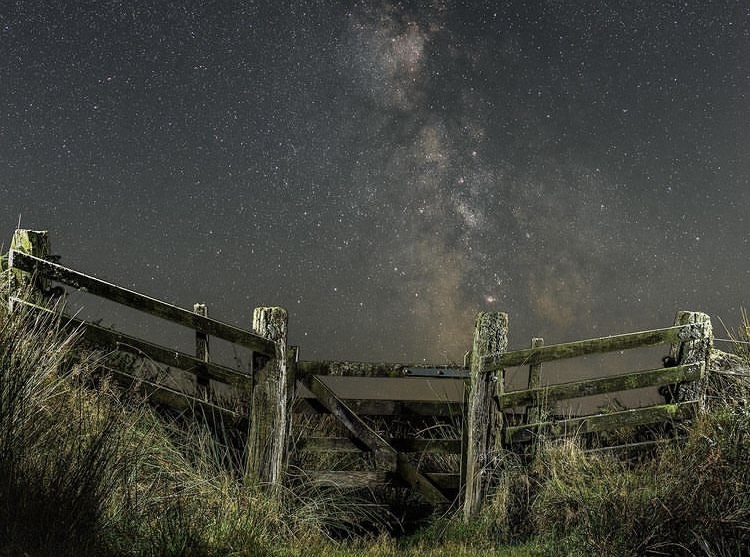This is an outdoor photograph showcasing a serene, open farm setting. At the bottom, the ground is covered in long grass, intermingling green and brown hues. A weathered wooden fence, showing shades of gray and green, crisscrosses the grassy terrain, some sections appearing to lean and collapse, suggesting disrepair. Above the fence and grass, the vast sky unfolds, revealing a spectacle of countless white stars and part of the Milky Way galaxy, creating space clouds that add depth to the night sky. The backdrop sky has a light grayish tint, likely illuminated by the multitude of stars. The scene is void of any animals or people, evoking a tranquil and untouched rural atmosphere, where the only presence is the celestial display overhead, making the farm appear peaceful yet brimming with the silent beauty of the cosmos.